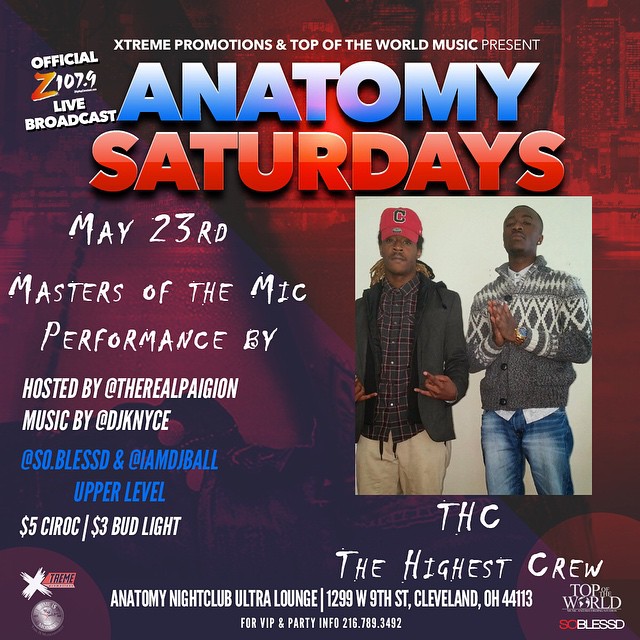This vibrant digital advertisement, displayed in a busy blue and red color scheme, promotes an exclusive VIP party event called "Anatomy Saturdays" at Anatomy Nightclub Ultra Lounge, located at 1299 West 9th Street, Cleveland, Ohio. Happening on May 23rd, the event features a live, captivating "Masters of the Mic" performance by THC, The Highest Crew, a duo of stylish African American men likely in their 20s to 30s. They strike compelling poses, one making horn signs with his hands and the other donning a fancy sweater, looking directly into the camera. The event is hosted by The Real Pae Gien with music provided by DJ KYNYCE at So Blessed and IMDball Upper Level. Drink specials include $5 Cirque OC and $3 Bud Light. For VIP and party information, attendees can contact 216-689-3492.